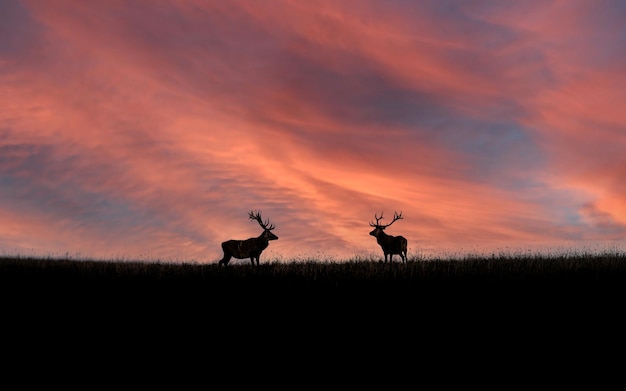In this captivating photograph taken at dusk, the vibrant sky steals the show with its stunning palette of oranges, pinks, and blues, creating an enchanting backdrop that blends beautifully with billowy clouds tinged in twilight hues. Silhouetted against this mesmerizing canvas are two majestic male moose, locked in a tranquil yet curious stance as they face each other. The moose on the left, displaying a prominent set of antlers, seems to gaze directly at his counterpart, whose antlers are visible from a different angle, enhancing the visual symmetry. They stand on a dark, grassy expanse at the bottom quarter of the image, where delicate blades of grass wisp upwards, grounding the scene in a tranquil, natural setting. The contrast between their dark forms and the radiant sky highlights the timeless beauty and serene mystery of the wilderness.